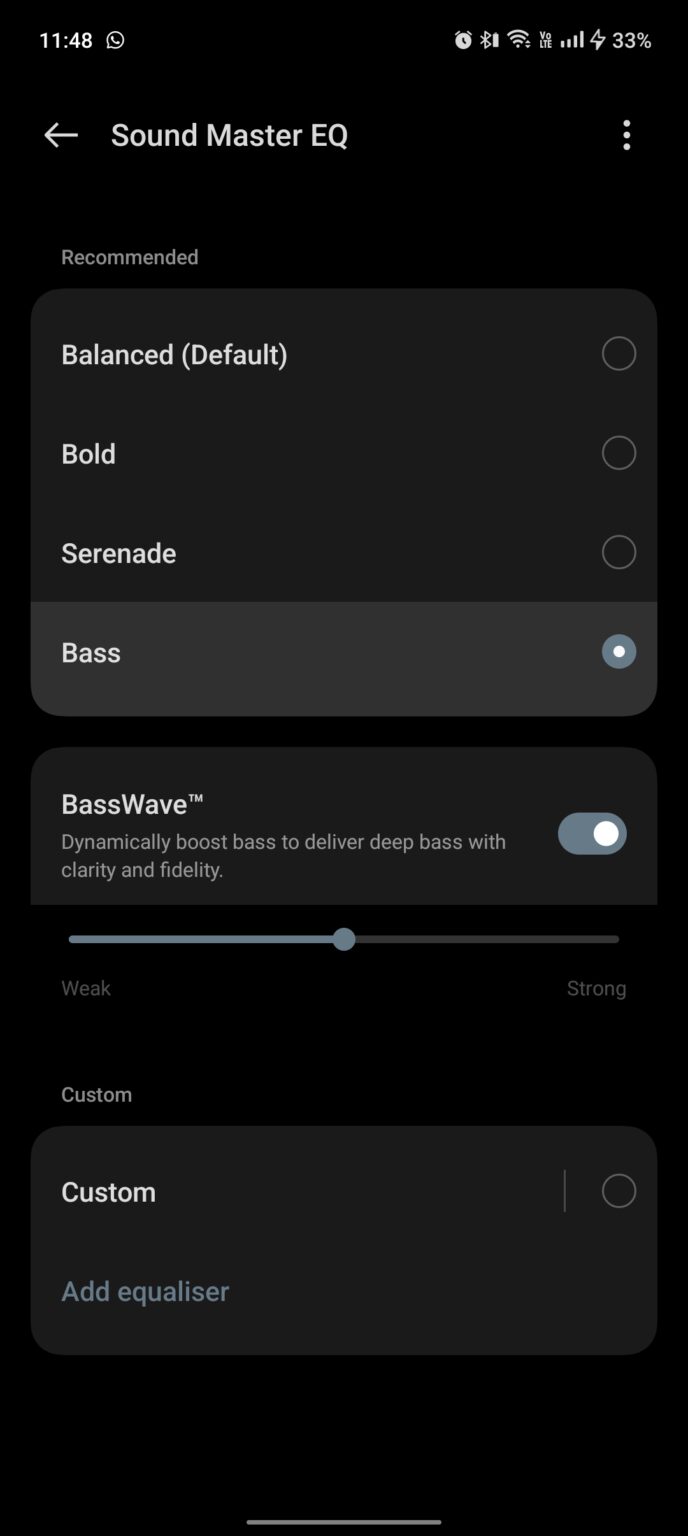Here is a refined and detailed caption for the described screenshot:

---

**Screenshot of SoundMaster EQ on a Phone Interface:**

The screenshot displays the SoundMaster EQ app on a smartphone. The overall interface features a sleek black background with contrasting white text. 

- **Top Bar Information:**
  - **Time:** Displayed in the top-left corner, showing 11:48.
  - **Icons (Left to Right):**
    - Analog clock icon.
    - Bluetooth symbol.
    - Wi-Fi signal strength indicator.
    - Settings icon represented by vertical bars.
    - Battery life indicator showing 33%.

- **Header Section:**
  - **Left Arrow:** Located below the top bar, pointing left, typically used for navigation.
  - **Title:** The application title "SoundMaster EQ" is centrally positioned.
  - **Menu Icon:** Three vertical dots are situated on the far right, indicating additional options.

- **Section for Presets:**
  - **Recommended Label:** Light gray text labeled "Recommended" is on the left.
  - **Default Preset:**
    - A charcoal gray rectangle containing the text "Balanced (Default)" in white.
    - A circular selection oval positioned to the right.
  
- **Additional Presets:**
  - **Bold:** Label with a circular selection oval on the right.
  - **Serenade:** Label with a circular selection oval on the right.
  - **Bass:** Label with a circular selection oval on the right.

- **Special Preset:**
  - **Bass Wave:** Label with the accompanying description "Dynamically Boost Bass to deliver deep bass with clarity and fidelity." 
  - **Adjustment Bar:**
    - The bar is positioned underneath the description, with the indicator set to the middle.
    - The labels "Weak" on the far left and "Strong" on the far right.

- **Custom Settings:**
  - **Custom Label:** Located below the bar.
  - **Custom Preset Button:** A gray rectangle with the text "Custom" inside.
  - **Add Equalizer Option:** The final option at the bottom, labeled "Add Equalizer."

The design is minimalistic yet functional, catering to users who seek to customize their audio experience through various presets and settings.

---

This caption now presents the information in a clear, structured manner while incorporating all details from the original input.